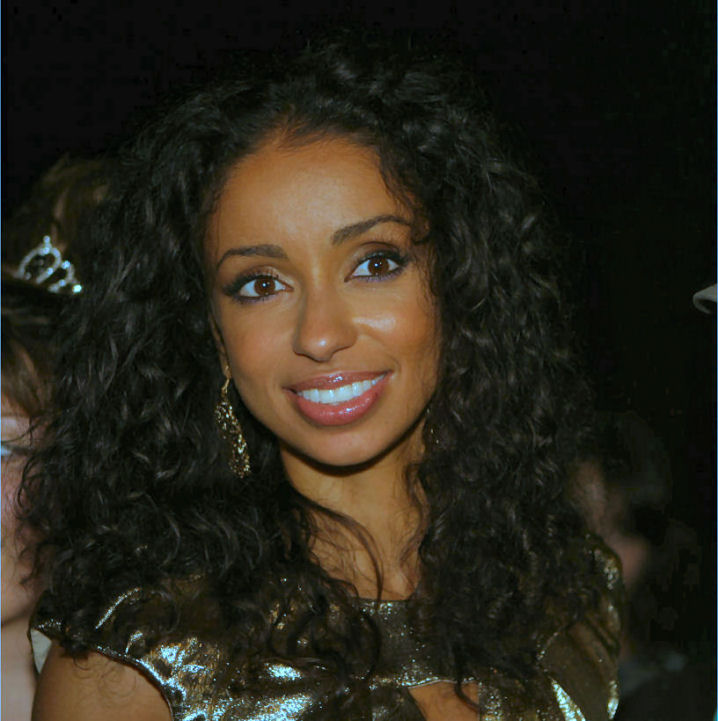The photograph features a woman with a medium brown complexion, smiling radiantly, displaying her white teeth. Her face is framed by shoulder-length, shiny, dark curly hair. She has rich chocolate brown eyes that are directed to the right side of the photograph while her face is oriented forward and her torso slightly turned to the bottom right. Her attire includes a reflective gold sleeveless dress with a distinct triangular cutout on the chest. Complementing her ensemble, she wears large dangling gold earrings. The background, primarily black, emphasizes her as the focal point of the image. You can faintly discern various out-of-focus figures behind her. On the left side, a woman is visible with a silver tiara perched on her medium dark hair, looking to the left. To the right, part of a grey hat brim can be seen peeking into the frame.